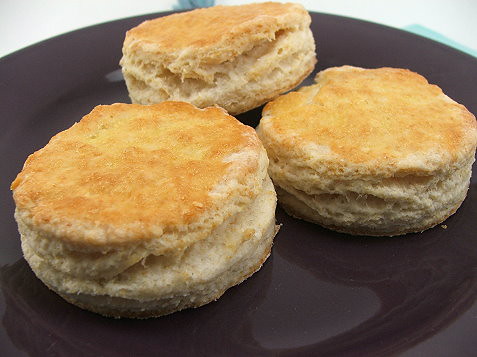The image captures a close-up photograph of three buttermilk biscuits arranged in a triangular formation on a shiny black plate, which sits on a barely visible white surface. The biscuits, which appear to be the fluffy, layered kind you get from a Pillsbury Doughboy tube, are nicely browned on top and reveal their soft, peel-apart texture. The front two biscuits sit side-by-side while the third is slightly elevated in the back, showing off the laminated layers that make them easy to pull apart. The camera's proximity allows for a detailed view of the biscuits' texture, highlighting their golden tops contrasted with the light, baked dough beneath.